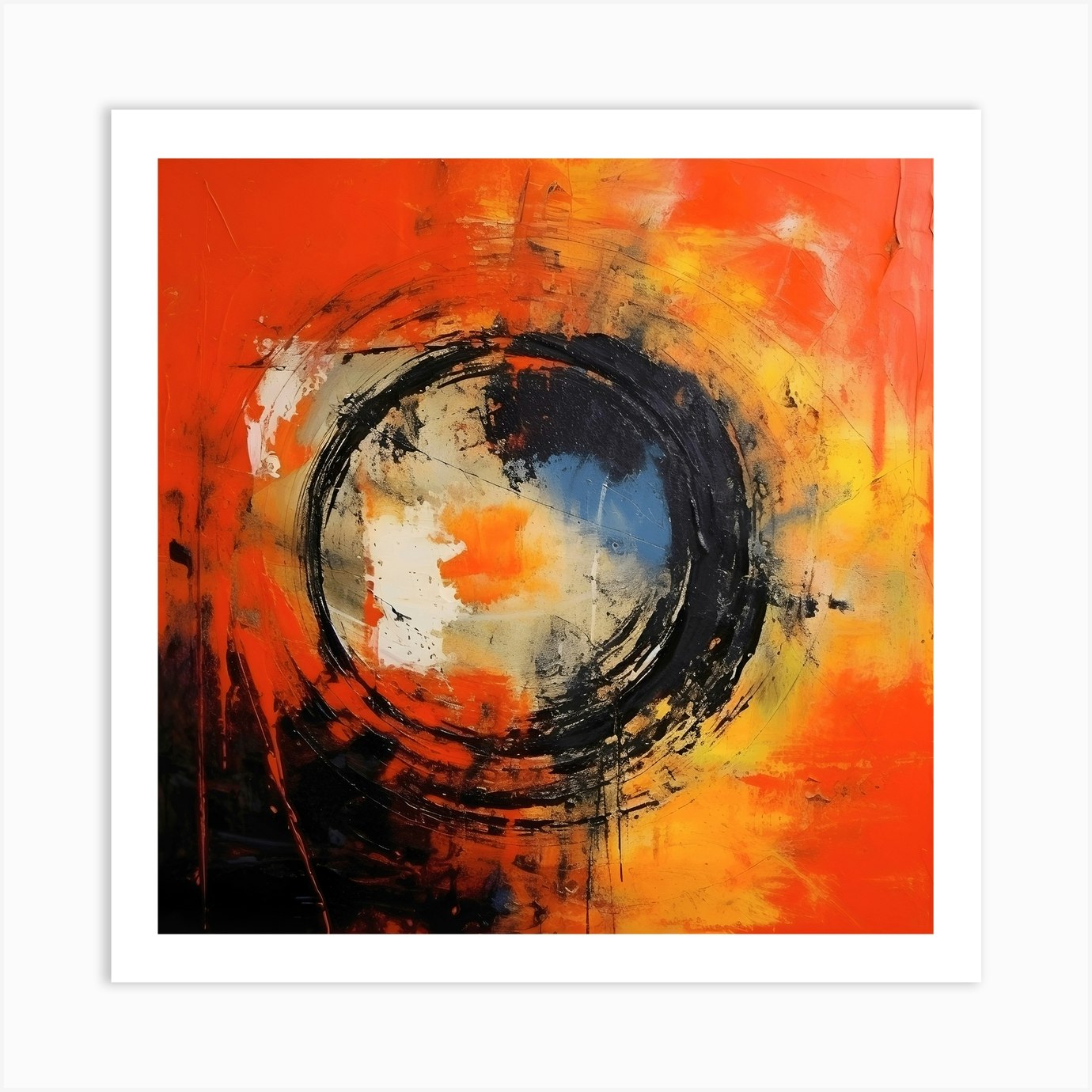This abstract oil painting is encased in a wide white frame and matting. The artwork itself is square, bursting with vibrant colors. Dominantly reddish-orange hues engulf three quadrants of the canvas, while the lower left corner is a stark, deep black. At its heart, the painting features a smudged yet distinctly circular swirl in the center, which evokes a sense of a paint can's top swirling with mixed colors. The circle's sketchy black outline encompasses a myriad of colors including blue, light brown, yellow, orange, white, beige, gray, and more reddish tones. Streaks and small shreds of red paint and yellow tints spiral outwards from this central swirl, creating an impression of dynamic movement, as though the colors are spinning off into the surrounding space, blending into the dominant red and black backdrop. Despite its abstract nature, which might not appeal to everyone, the intricate details and vivid palette make it a unique and striking piece of art.